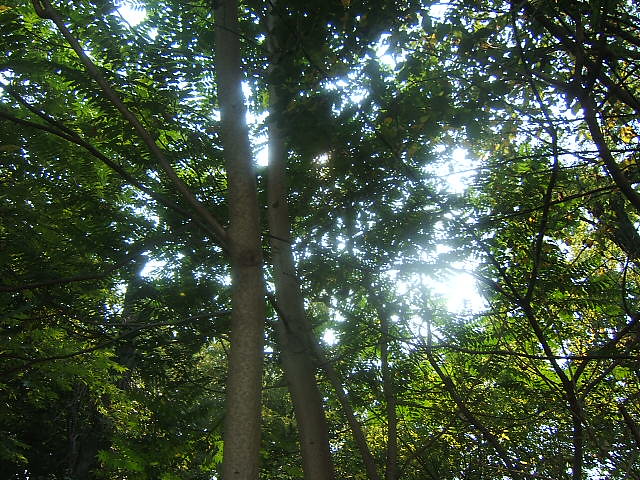The image features a stunning low-angle photograph of the woods, capturing the canopy of tall, slender trees with branches extending in all directions. The trees, appearing to reach heights of 40 to 60 feet, are predominantly green with interspersed shades of yellow. The sky peeks through the dense foliage, creating a mosaic of blue and white in the gaps between leaves. Sunlight filters through the canopy, illuminating the leaves and casting a radiant glow that highlights the various greens and yellows. The main trees in the photo have light tan bark and are notably tall but not particularly thick. The overall composition of the photograph beautifully showcases the intricate interplay of light and nature, emphasizing the lush greenery and the tranquil beauty of the wooded scene. There are no people, animals, or birds in sight, keeping the focus purely on the natural splendor of the trees and their leaves against the sunny sky.